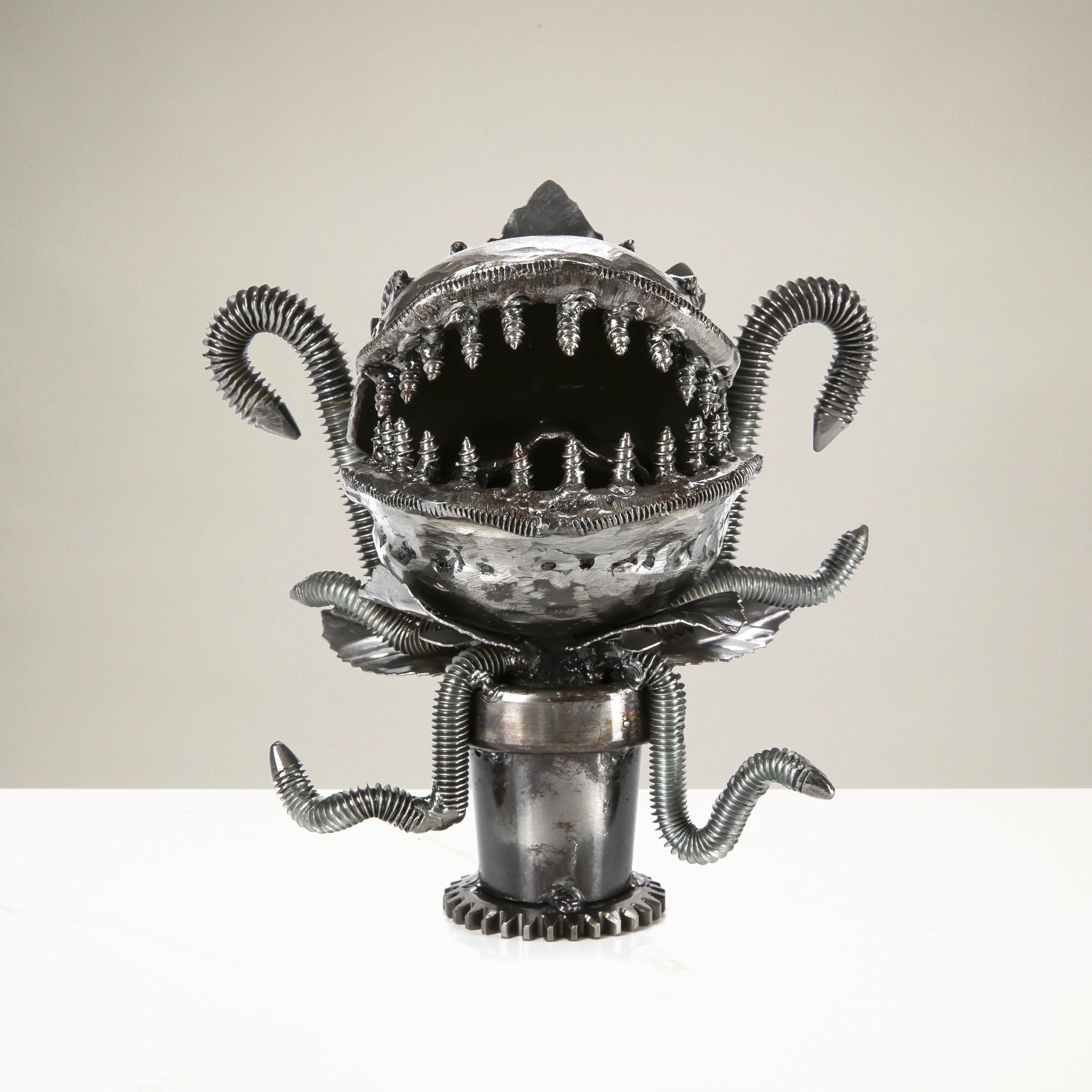The image depicts a striking black and white photograph of a shiny, silver metallic sculpture. The sculpture, which resonates with the character "Audrey" from Little Shop of Horrors, is a monstrous, flower-like creation. It sits atop a round, cylindrical base adorned with small spikes, resembling a coaster. Emerging from this base are six earthworm-like tubes, with two extending downwards, two upwards through the center, and two curving to the right.

Dominating the top of the sculpture is a large, round shape featuring an enormous mouth with a curved opening. This mouth is equipped with teeth made from small metal screws, enhancing its menacing appearance. The entire piece exudes an eerie, yet captivating artistic homage to the man-eating flower, Audrey. The background is simple black and white, emphasizing the sculpture's intricate metallic details and gleaming surface.